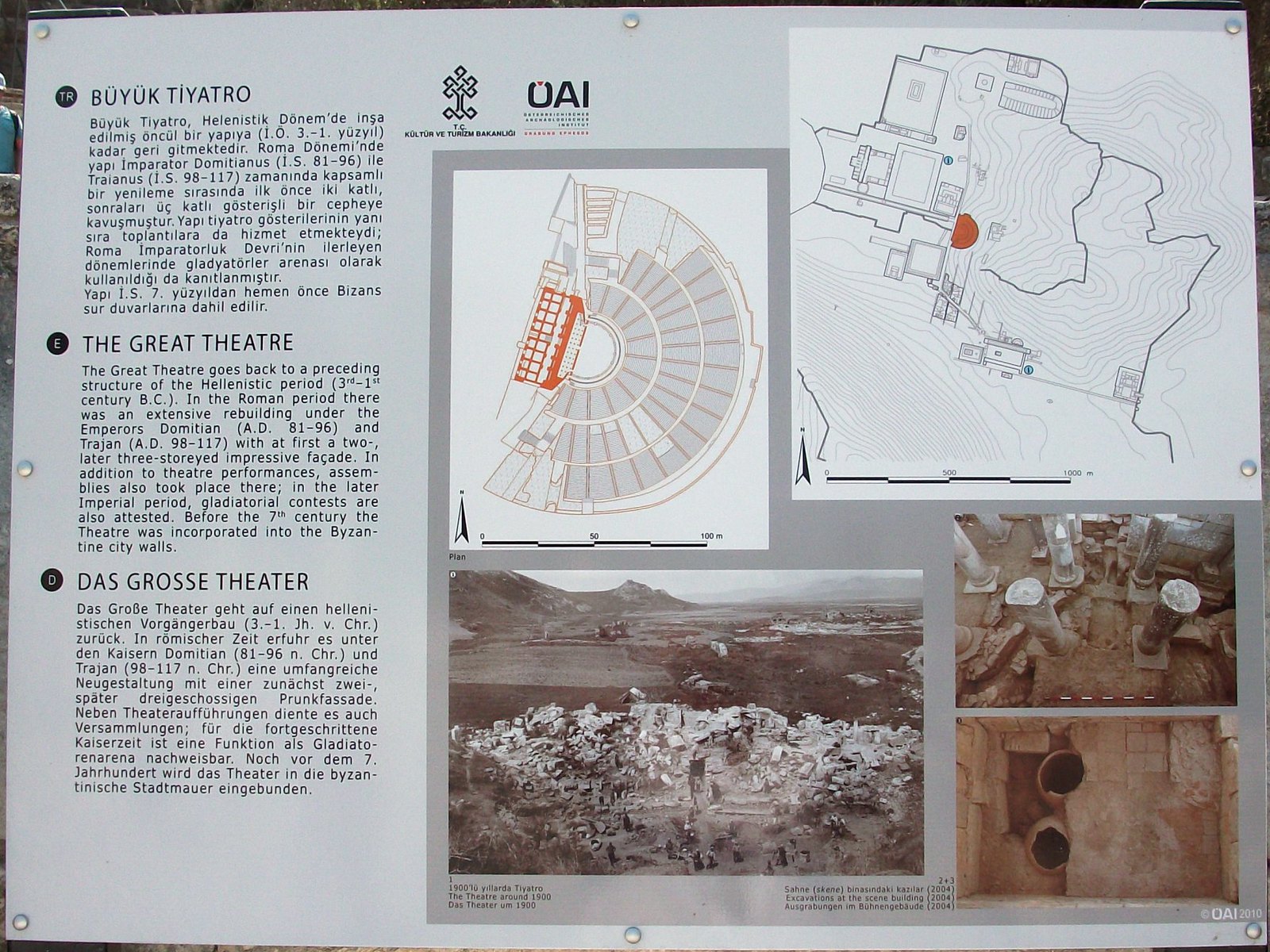The image shows a detailed signboard describing the Great Theater, an ancient landmark of significant architectural and historical importance. Central to the sign is a seating chart of the theater, with the stage depicted in orange and semi-circular seating radiating outward. To the right, an aerial diagram illustrates the theater's geographic location, set against a hilly plateau. Below this geographic map are three photographs depicting architectural ruins: one shows remnants of an excavation site, another captures ancient columns from an overhead view, and the third features the ruins with distant mountain ranges in the background.

The left side of the sign presents the information in three languages: in English, as "The Great Theater," in German, "Das Große Theater," and in what appears to be Turkish, "Büyük Tiyatro." The descriptions explain the theater's historical context, dating back to the late 3rd and early 4th century BC during the Hellenistic period, with significant extensions during the Roman period under Emperors Domitian and Trajan.

At the top of the sign are the letters "UAI" in blue on a white background, accompanied by an unspecified symbol. The text also discusses the underground construction features of the theater, adding to the understanding of its engineering marvels. The sign essentially serves as a comprehensive guide to the theater's historical development, architectural layout, and excavated remains.